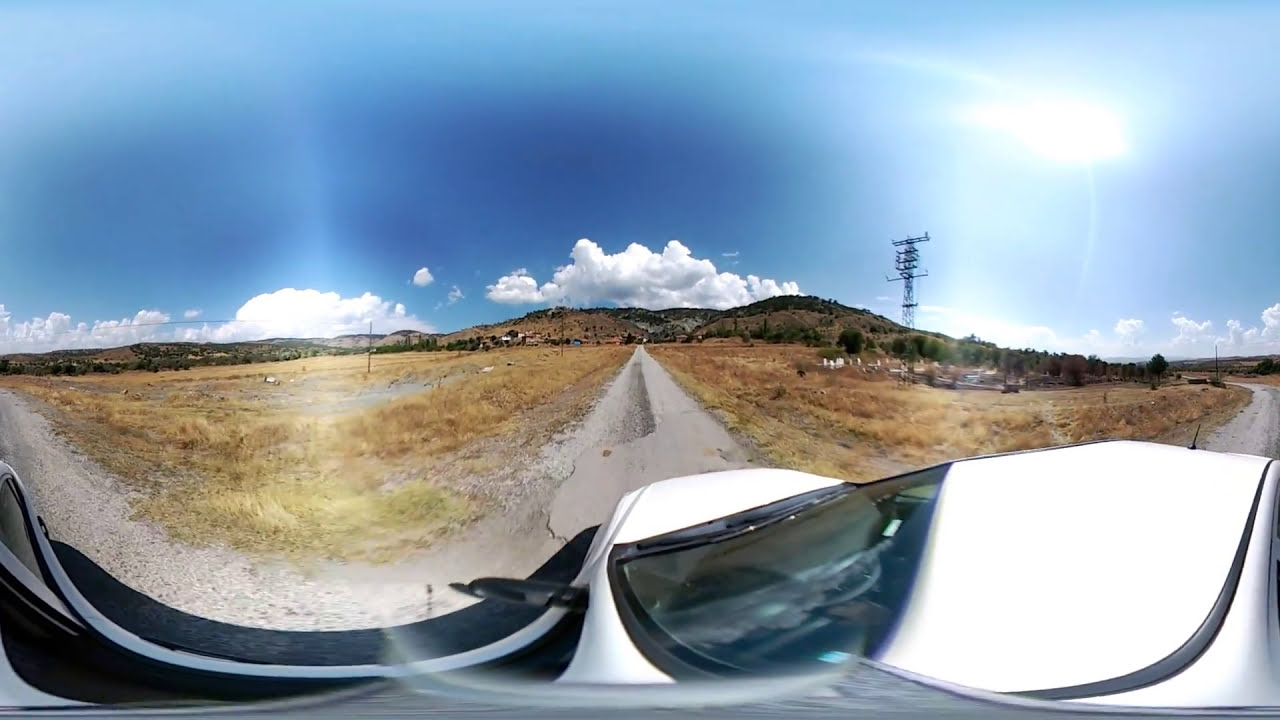An outdoor image captured via a GoPro helmet camera or a Fish Eye lens, possibly through the windshield of a white vehicle. This mid-to-late afternoon scene showcases a sweeping blue sky punctuated by low, puffy white clouds. The upper 40% of the picture features a skyline backdrop with brownish-green low hills, extending across the horizon from left to right. Dominating the right side of the image is a tall, possibly communication tower, potentially with some buildings around its base. 

The foreground reveals a central, poorly maintained dirt road in grayish tones that bifurcates and curves out of the frame, flanked by fields of dry, brownish-green vegetation. The road surface alternates between asphalt and gravel. The lower part of the image prominently shows the front section of the vehicle, identifiable by its white color with black and gray accents. There might also be a greenish tint visible in the vehicle's windows, suggesting the shot might be taken through them.

Overall, the scene offers a panoramic view of a desolate, dry landscape traversed by a solitary road, with the entire composition suggesting an empty, rugged, and serene environment.